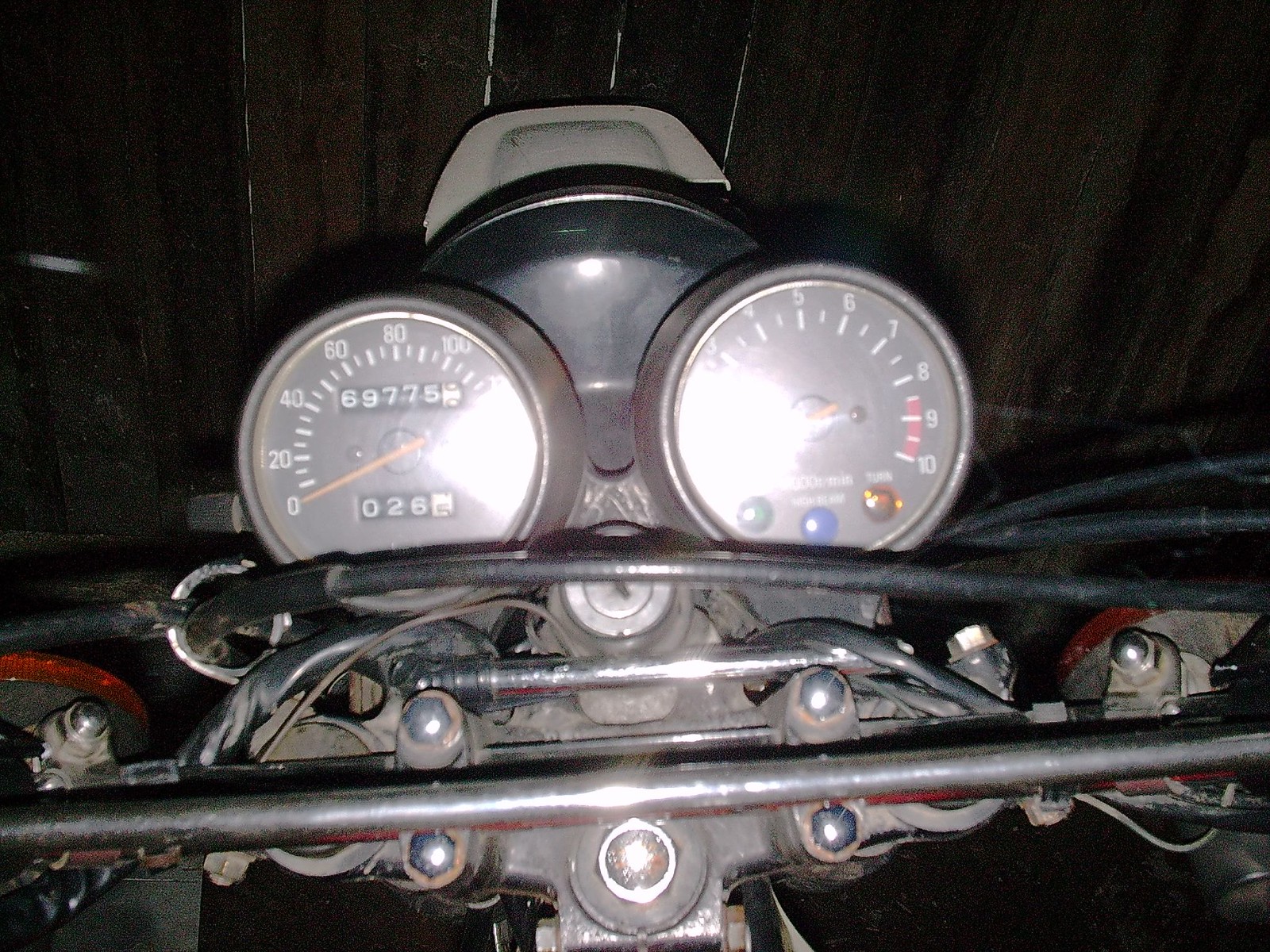The image showcases the speedometer and tachometer of a motorcycle, reflecting a high odometer reading of 69,775 miles, indicating extensive use. The trip meter displays a recent journey of 26.5 miles. The speedometer needle rests at zero, indicating the motorcycle is stationary, and the tachometer needle is also at rest. A bright light obscures some of the tachometer and speedometer numbers. Just below the instruments, a keyhole hints at its central locking mechanism. The handlebar, partially visible, stretches across the composition, with a headlight subtly shining ahead. The instrument cluster is primarily black, featuring white numerals and orange needles. Additionally, some green, blue, and amber indicator lights pepper the tachometer, adding a splash of color. The entire scene is set against a black backdrop, suggesting it might be nighttime. Various cables snake along the handlebar, blending into the predominantly monochrome color scheme, punctuated by the vibrant instrument lights.